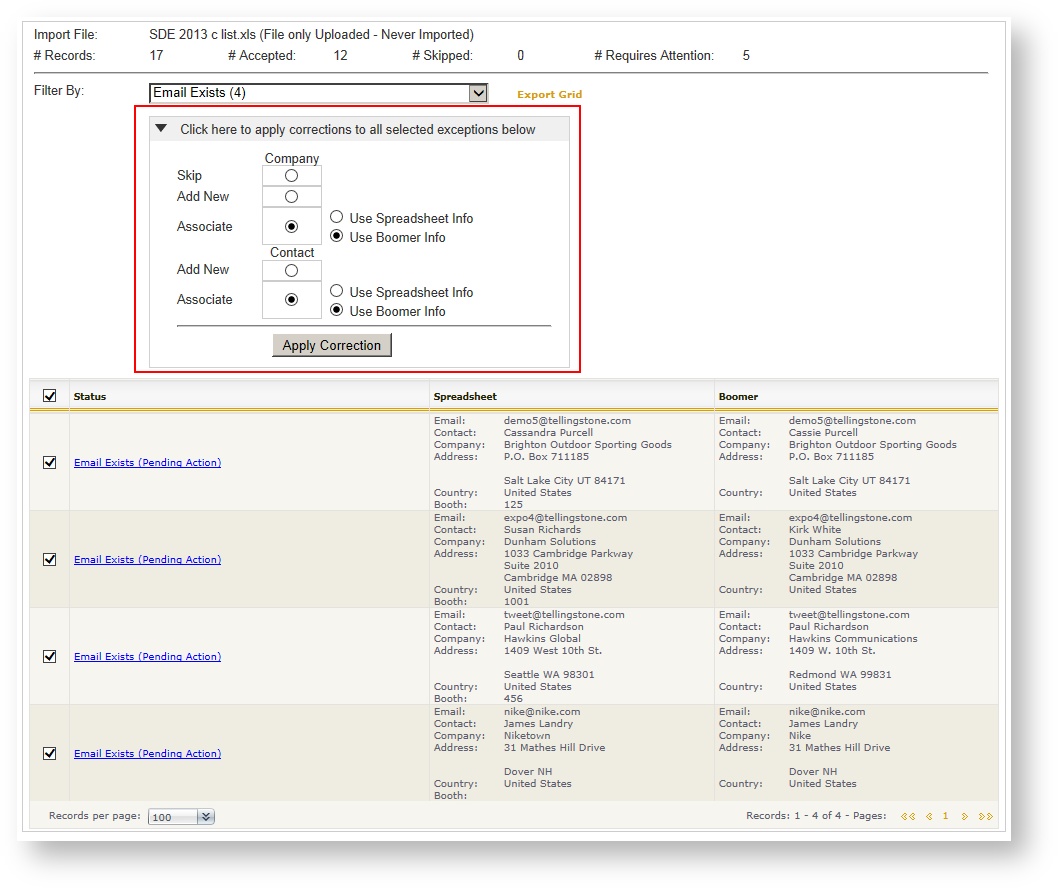On a white background, the image features an interface consisting of various sections and options related to file import and record management. At the top, there are filters and status indicators for imported files, represented by a hashtag (#) symbol, with the following details:

- Total records: 17
- Accepted: 12
- Skipped: 0
- Requires Attention: 5

A red rectangle highlights a box with an action button labeled "Click here to apply corrections to all selected expectations below". 

Below this, the interface presents several organizational fields. There are options to add a new associate, and a section on associates, some of whom are shaded to indicate selection. Specifically, it includes:
- "Company" 
- "Add new associate"
- "Associate" with shaded or selected circles

To the side, there are options to use information from a spreadsheet or a system referred to as "boomer", with "Use boomer info" being shaded. This section is duplicated with identical choices of using spreadsheet info or boomer info, every time with "Use boomer info" preselected. 

A grey rectangle button labeled "Apply Correction" is prominently displayed. 

Towards the bottom, the layout resembles a spreadsheet with several columns, checkboxes, and status indicators. All checkboxes within this section are checked, and the columns are labeled:
- Status (examples include "Email exists" and "Pending action")
- Spreadsheet
- Boomer

The status indicators and action buttons are highlighted in blue, bringing attention to required interactions within the interface.